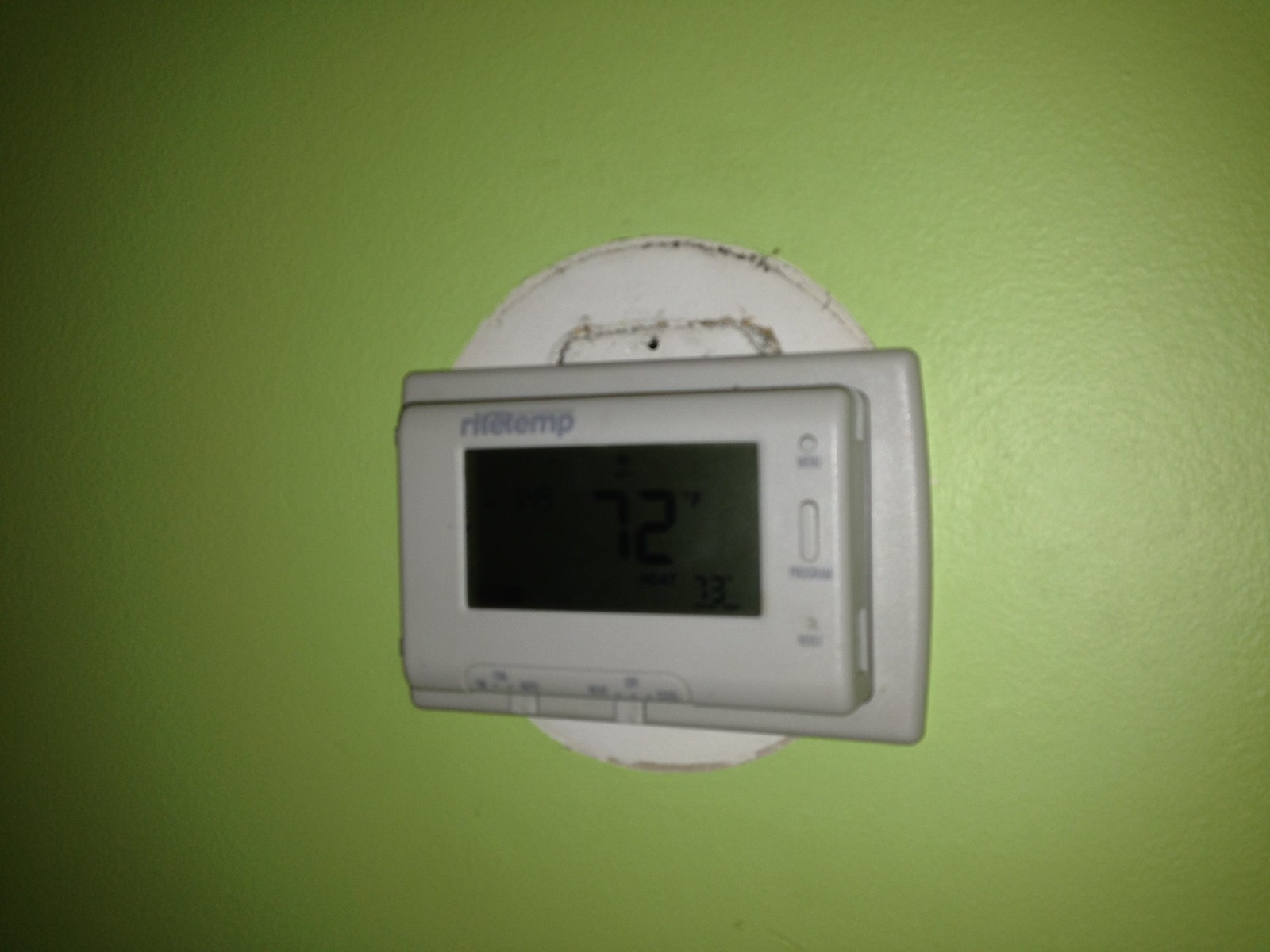The photograph captures an outdated, slightly dirty thermostat mounted on a light green semi-gloss painted wall. The paint reflects light, revealing the characteristic subtle bumps of the finish. There's a distinctive circular outline around the thermostat, suggesting that a circular white plastic plate once surrounded the device but has since been removed, leaving the white backdrop of the original wall color exposed. This outline is accentuated by a layer of dirt, particularly more concentrated at the top and bottom of the circle.

The thermostat itself is a rectangular device with a light gray casing, prominently branded with "RITE-TEMP" or a similar name. It features a digital display with black lettering, showing a current temperature of 72 degrees. To the lower right of this main reading, a slightly smaller display reads 73 degrees with a degree symbol. To the right side of the thermostat, there are several buttons, although the labels are indistinguishable in the photo. Additional adjustment controls are located towards the bottom of the device.